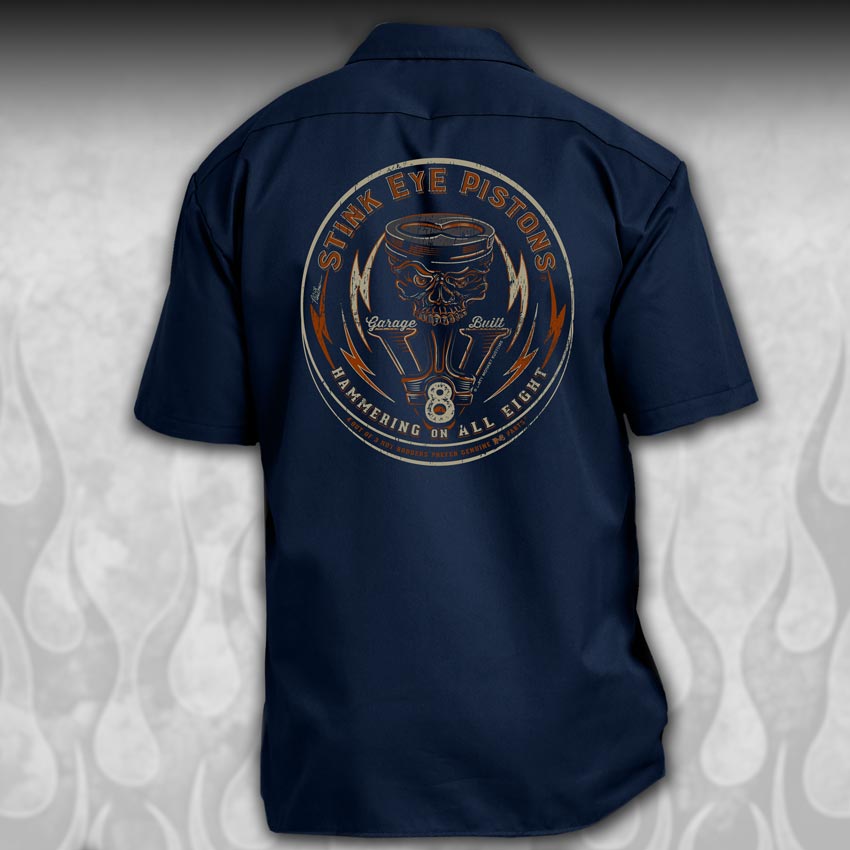The image features the back of a navy blue short-sleeved, button-up work shirt set against a unique background with a beige, marbled look that transitions into gray flames towards the bottom. The shirt prominently displays a circular graphic in the center. In striking red letters, the top of the circle reads "Stink Eye Pistons." Below that, a stylized V8 engine with a partially visible skull as its centerpiece is depicted, complemented by three white and red lightning bolts on either side. The phrase "Garage Built" is inscribed on the engine heads. Near the bottom of the circle, the text "Hammering on all 8" is displayed, with the number "8" beneath it, all in light lettering. Additional text in orange is present but too small to be legible. The shirt's back is meticulously designed, highlighting a blend of automotive and rebellious themes.